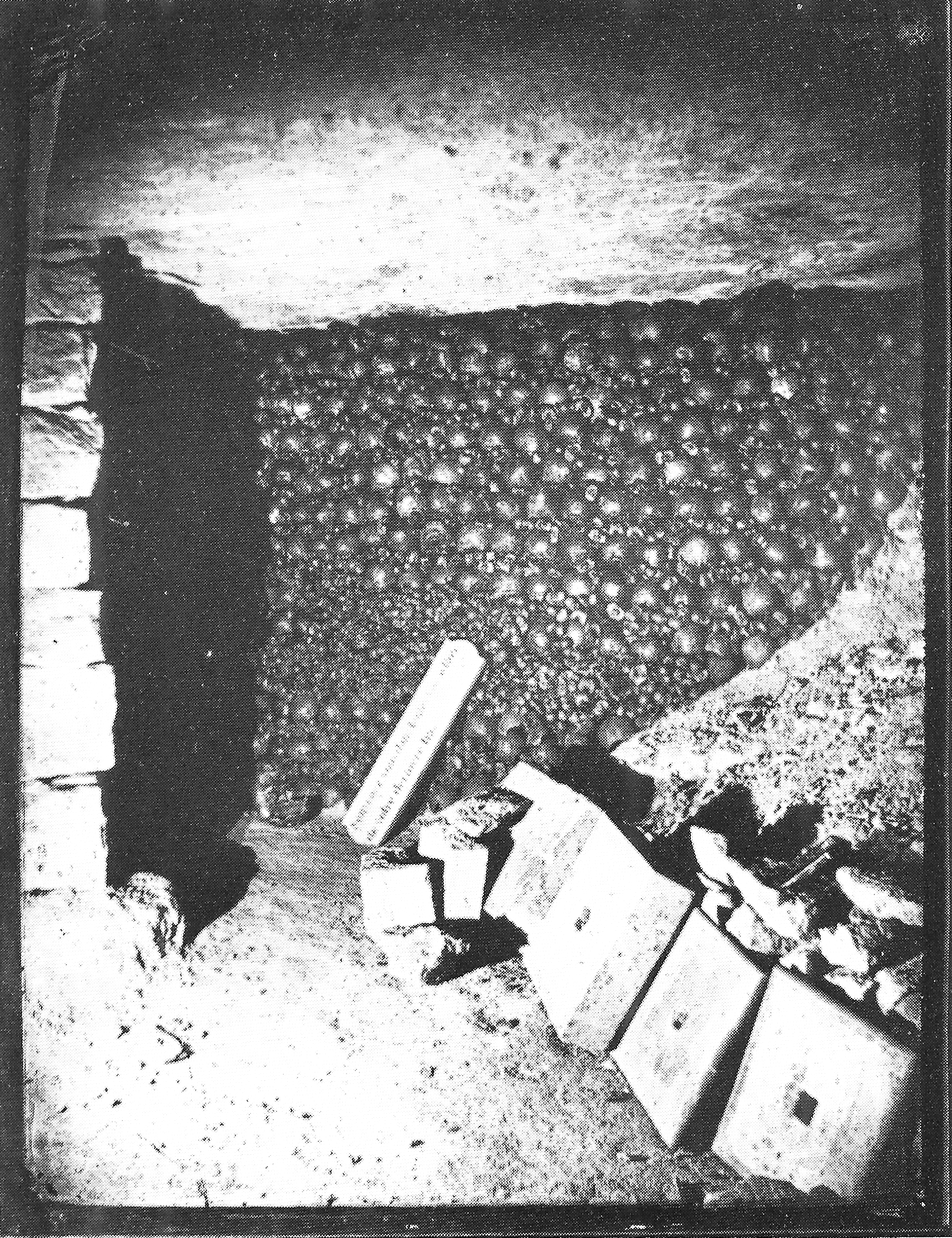The black and white photograph captures an underground scene, evoking the mystique of the Parisian catacombs. To the bottom right of the image lie square bricks, each featuring a distinct square hole at their center, neatly arranged on the stone floor amidst rock and debris. The left side of the scene is dominated by a partially destroyed brick wall, with bulbous shapes protruding from its structure, resembling an array of skulls. Scattered around the floor are fragments of concrete and rubble, alongside a piece with indiscernible text in French, suggesting an ongoing excavation. The scene is partially illuminated by an unknown light source, casting an eerie glow over the desolate setting, all framed within a black border.